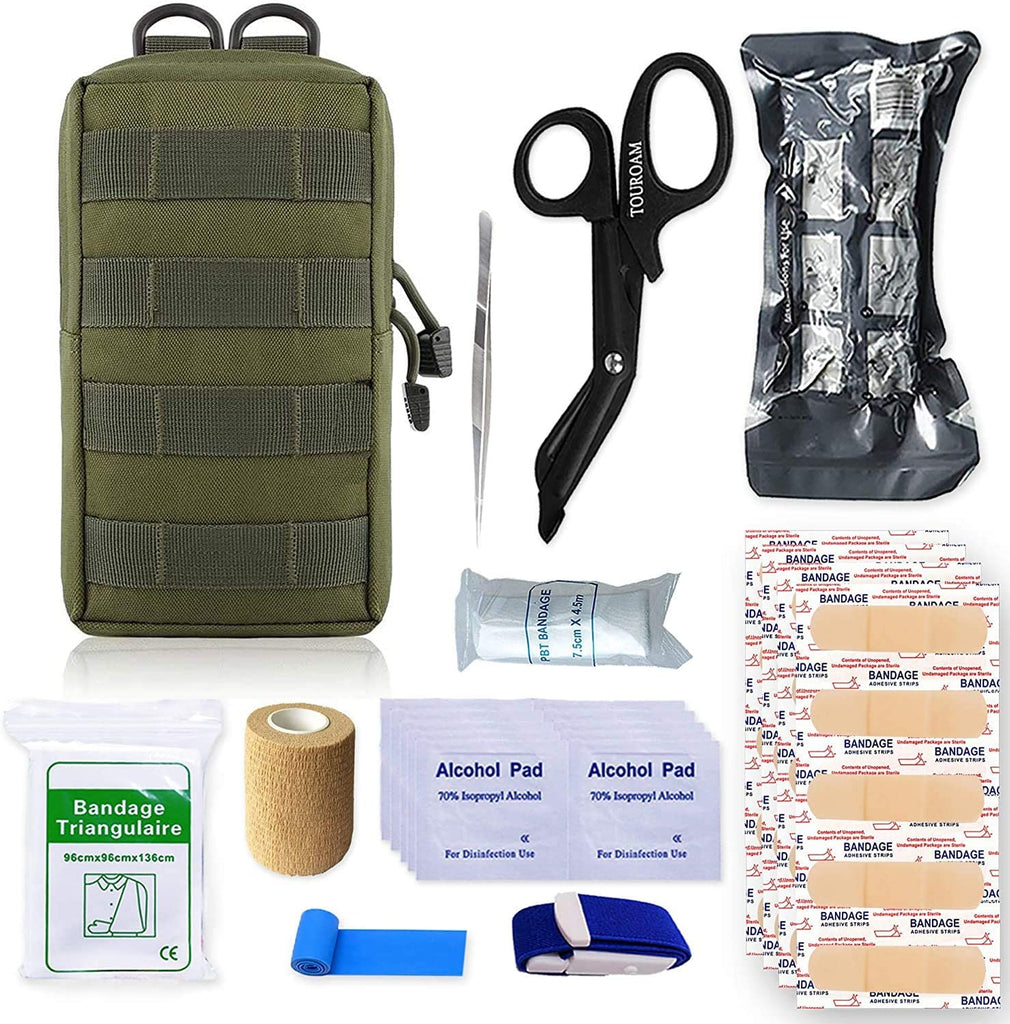The image depicts a meticulously arranged, deconstructed first aid kit against a white background. At the top left, there's an olive green, canvas bag with four gray straps and two top hooks, oriented vertically. To its right, a pair of silver tweezers with textured grips lie pointed downwards next to black Toroman scissors, which are slightly bent to the left. Beyond the scissors, a crinkly silver and gray package, which could be an emergency blanket, completes the sequence.

At the bottom left, a white rectangular package labeled "Bandage Triangular" in green text features an illustration of a headless torso with an arm in a sling. Nearby is a textured roll of tan gauze bandage, with a piece of blue tape slightly unfurled below it. Continuing rightward, a finger splint with white and blue details lies above a stack of alcohol pads in white packages. Adjacent to these items is a sheet of five tan bandages, backdropped by a label saying "Bandage" with red and dark blue accents.

This well-organized display showcases the variety of essential emergency items, emphasizing practicality and readiness for immediate use.